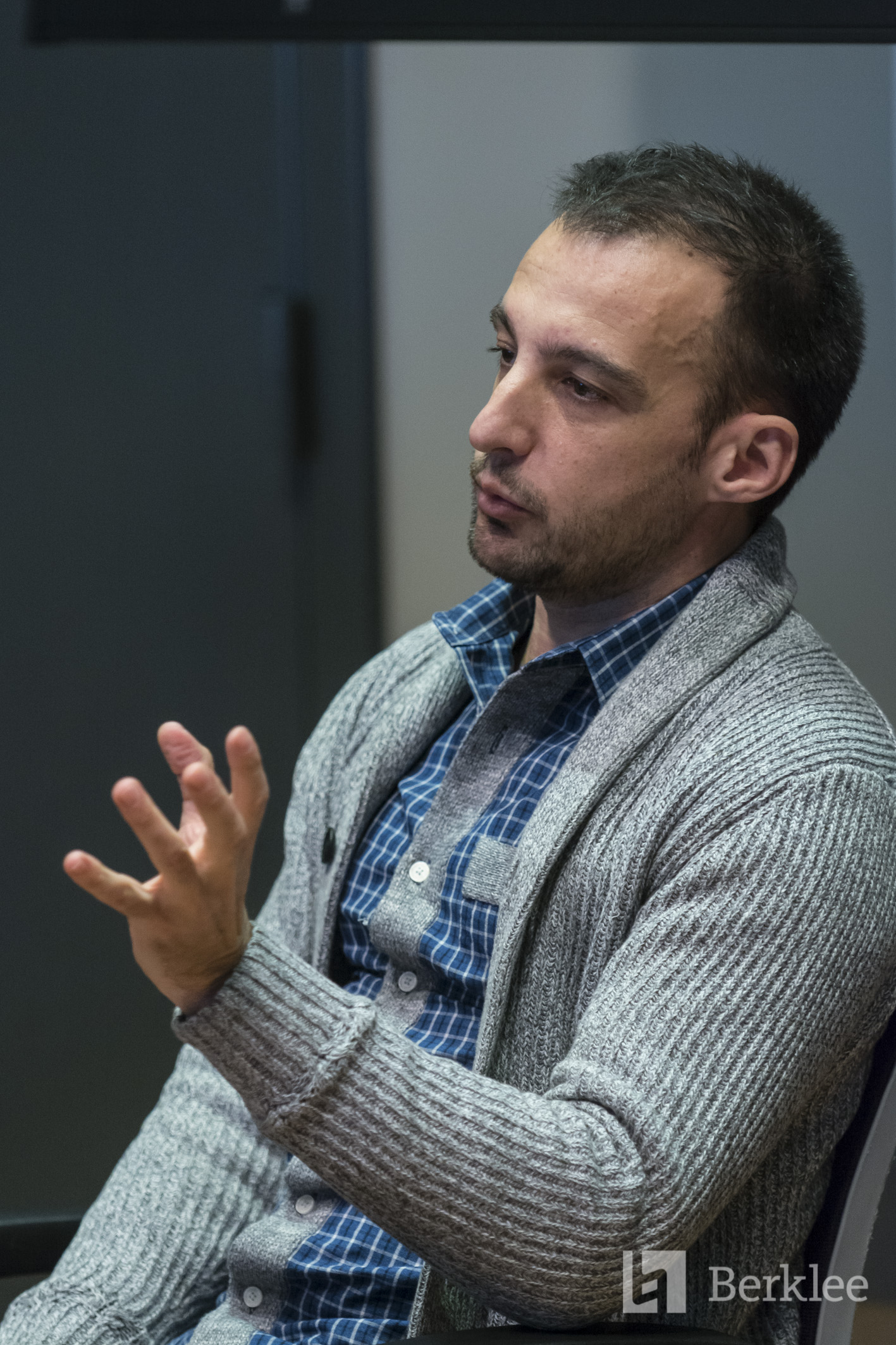This is a tall rectangular photograph capturing a man from the torso up, seated in what appears to be a classroom or auditorium. The man is slightly oriented towards the left while leaning back, with his head tilted mildly to the right. He is wearing a blue plaid button-up shirt bordered with gray around the buttons, layered under a gray sweater. The man's short, slightly balding brown hair frames a face adorned with a short mustache and stubble, which carries a serious expression. His left hand is raised and open, palm outward, while his right hand seems to rest on his lap. The background is blurry, displaying a monochromatic black and white wall. The chair he is sitting on has a visible curved spine and armrest, with an adjacent chair's edge visible in the lower right corner. Additionally, the bottom right corner of the image features a light gray square logo with the text "Berkeley" next to it.